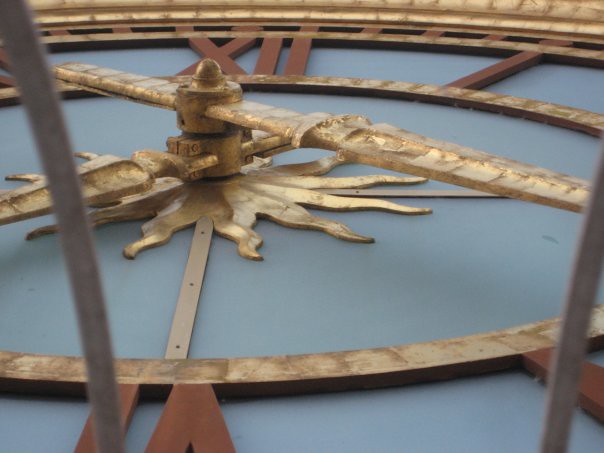This close-up photograph captures the face of a towering outdoor clock, viewed from a downward angle as if you're standing directly beneath it. Dominating the composition, the clock's details are magnified, showing only a portion of its face. The grand, golden hour and minute hands jut out prominently, with the minute hand seemingly pointing towards 5 and perhaps the hour hand towards 7. Surrounding them is a radiant golden sun emblem encircled by sun-like rays.

Encased in a glass backing, the clock's face features weathered Roman numerals, the "XII" and "I" clearly visible in a rusted brown hue, with the bottom part of the "VI" peeking in inverted. The background color of the clock face is a subtle, yet striking grayish-blue, highlighting the intricate design. The top edge of the clock is barely visible, hinting at an ornate outer ring also gilded in gold. The image is brightly lit, enhancing the vibrant contrast between the gold and the multi-toned background.